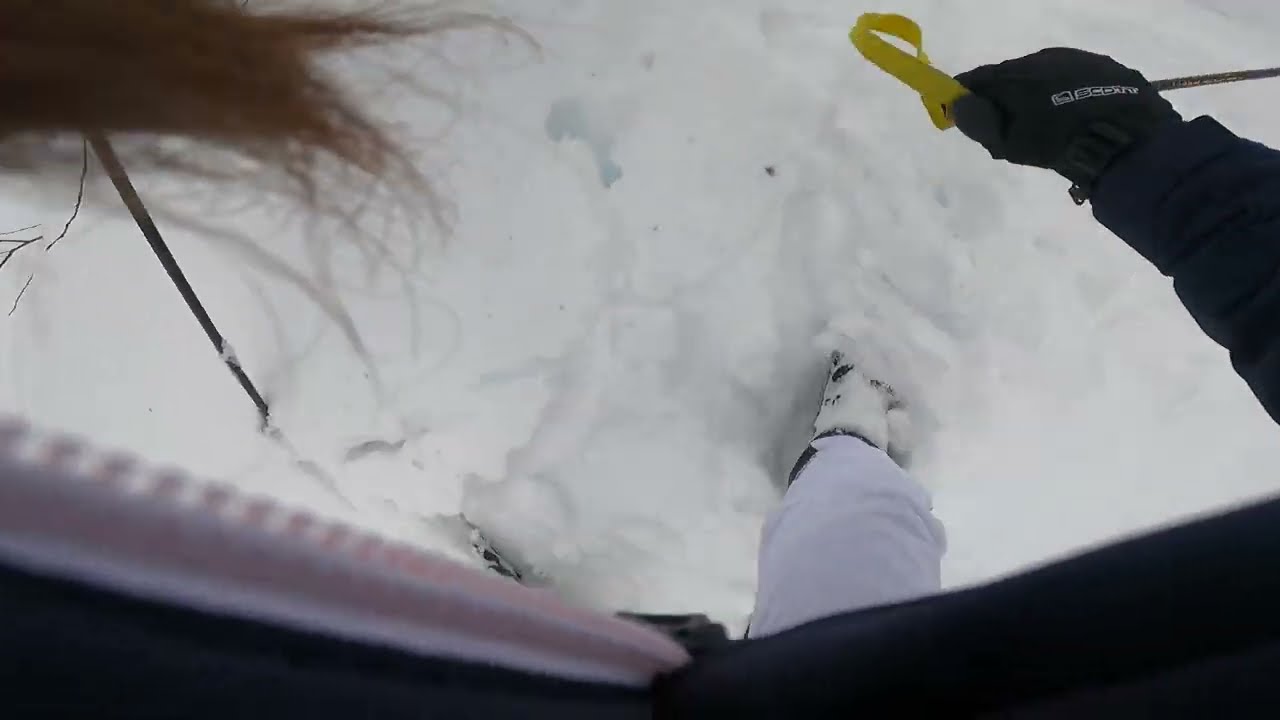The image is a horizontally aligned, rectangular close-up taken from a top-down perspective in bright, snowy conditions. In the upper right corner, a person’s right hand, clad in a black winter glove with white prints, holds a yellow strap or ribbon. Their jacket is dark blue or black, and they are wearing light purple or possibly white snow pants, with their right leg partially buried in thick, fluffy snow, making their shoe appear white. The foreground is dominated by this thick snow. In the upper left corner, strands of the person's brownish-red, wiry hair are visible, partially obscuring a yellow ribbon they may be holding in their left hand. There is also a visible white zipper. The scene suggests the person, possibly a female wearing a helmet or head-mounted camera, is engaging in an outdoor winter activity. There’s a brownish line in the snow that might be a crack or a tree branch, adding a subtle detail to the snowy setting.